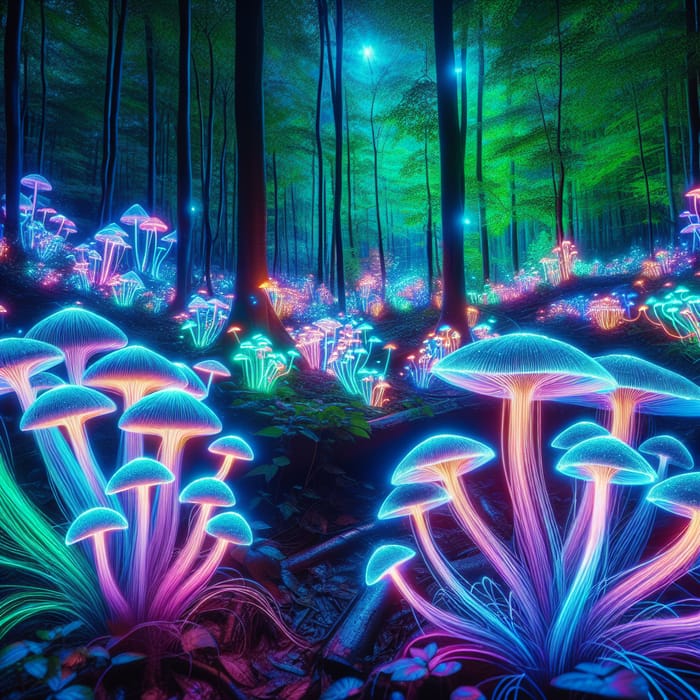This is a vibrant, color painting of an enchanting, imagined fantasy forest teeming with neon and fluorescent mushrooms. Covering the forest floor, the mushrooms glow intensely with blue and pink caps, with some featuring green, leaf-like structures emerging from their undersides. Closer to the viewer, there are two prominent groupings of mushrooms, each comprising 5 to 10 fungi. These luminous fungi exhibit a range of stem colors, from blue and pink to hints of orange and purple, some growing as tall as three to four feet. The forest backdrop features an array of narrow tree trunks and lush green foliage stretching off into the distance, where more mushrooms can be seen. Above, the sky is adorned with star-like lights shining through the treetops, complemented by the trees' green canopies. The scene is illuminated as if by invisible flashlights, enhancing the forest's magical and luminous ambiance.